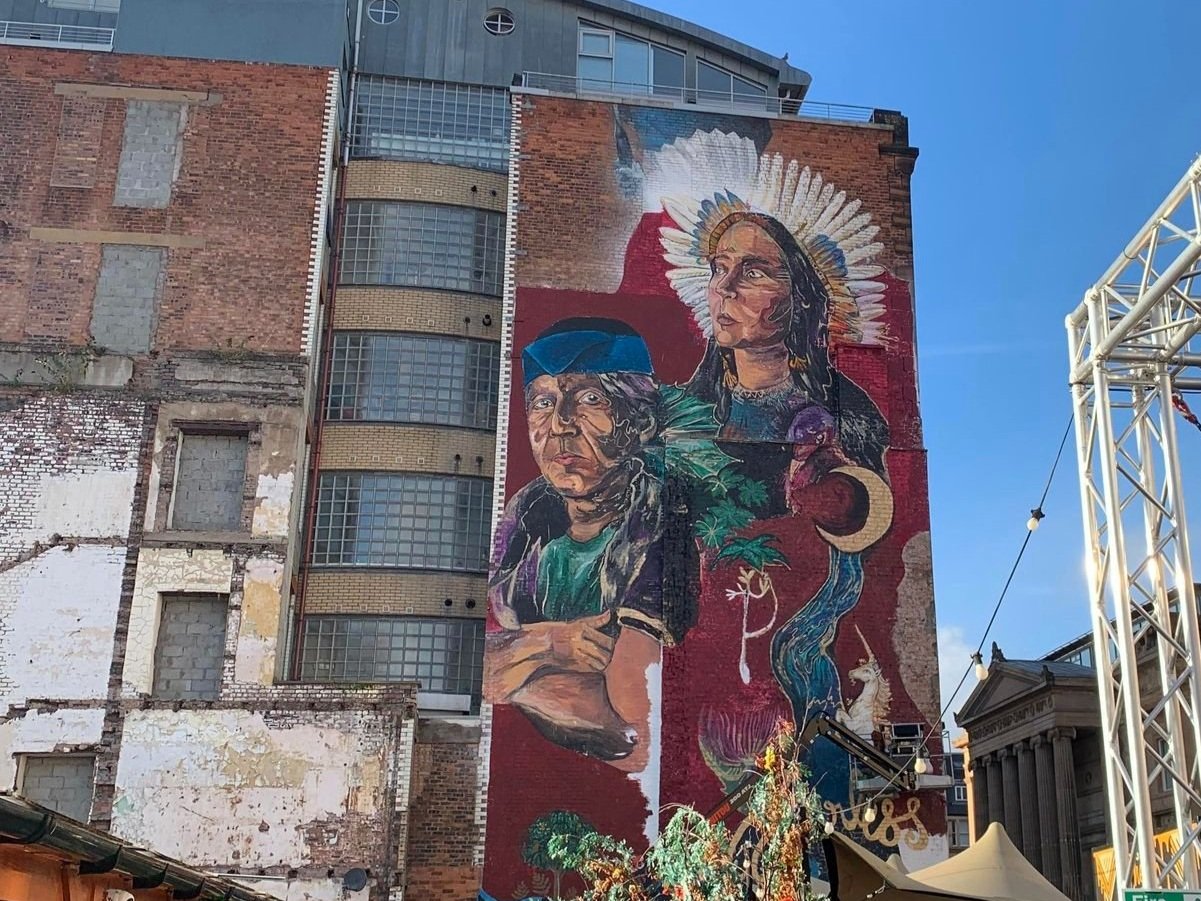The image depicts an outdoor scene featuring the side of an old, likely abandoned, five-story red brick building. The building is dilapidated, with some windows and doorways walled off or bricked over, and sections of white paint peeling from the lower areas. Metal scaffolding and string lights suggest possible stage use or maintenance activities nearby.

The highlight of the building is a striking mural that spans the height of the structure. The mural features two prominent figures, both Native Americans. The older gentleman on the left, perhaps in his 40s or 50s, is depicted with a solemn expression, gazing directly at the viewer. He wears a small blue hat, a green shirt, and a short-sleeved black jacket. His arms are crossed over his chest, and some green elements, possibly feathers, extend from his head.

To the right, a younger Native American, likely in their early 20s, is shown with long black hair and sporting an elaborate white feather headdress. This figure is gazing off to the side. Below the figures are additional artistic elements, including a crescent moon with a waterfall flowing from it and a unicorn, all set against a deep red background. There is no text present within the mural.